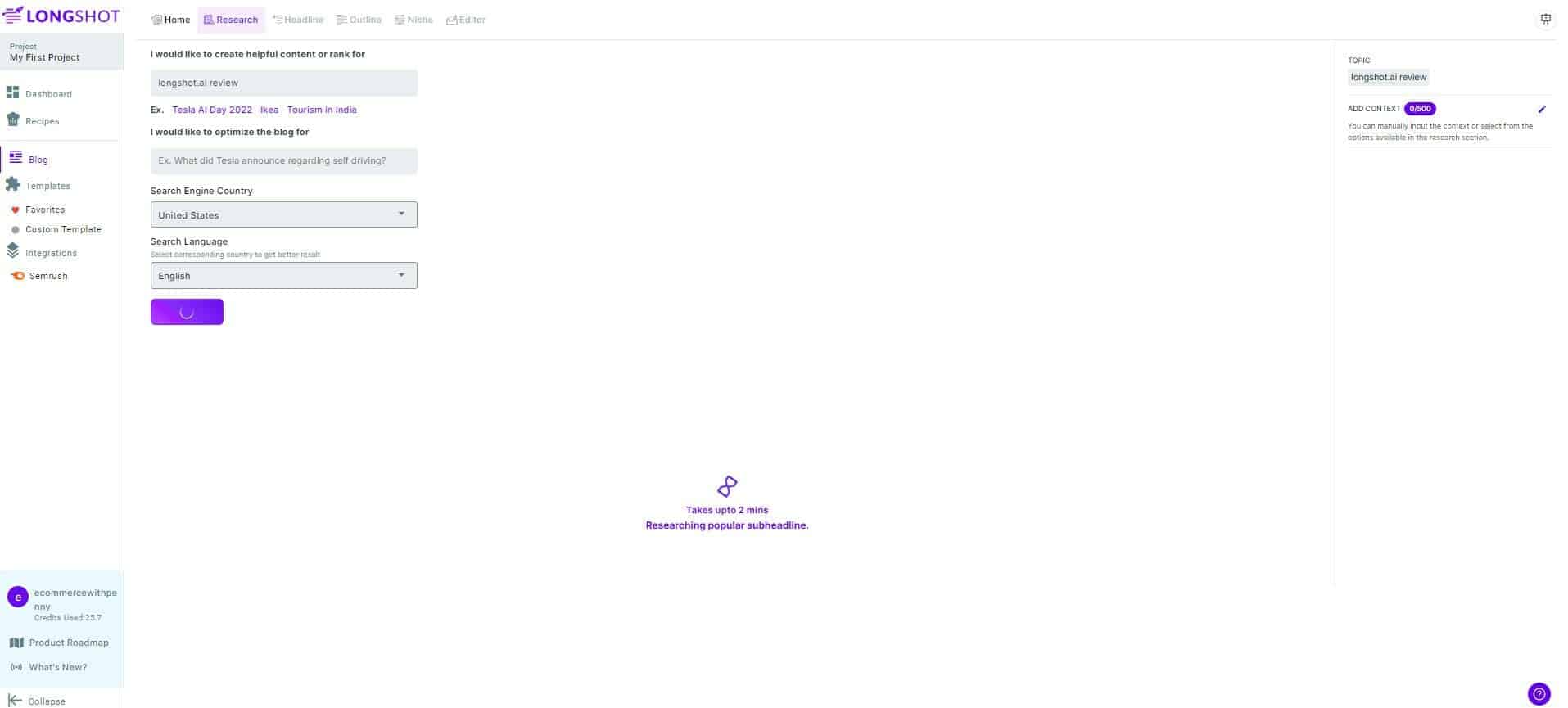Screenshot of a Website from a Computer Display:

The screenshot captures a website interface from a computer screen. On the top-left corner, a purple heading reads "Long Shot." Directly beneath it, a grey sidebar menu lists the following options, each accompanied by distinct icons (some in purple, green, red, and orange):

1. Project
2. My First Project
3. Dashboard
4. Recipes
5. Blog
6. Templates
7. Favorites (with a red heart icon)
8. Custom Template
9. Integrations
10. SEMrush

At the top of the screenshot, there is a horizontal navigation bar featuring the tabs: Home, Research, Headline, Outline, Niche, and Editor. Just below this bar, a text prompt states, "I would like to create helpful content or rank for," followed by a search option bar with the pre-filled text "longshot.ai review."

Directly under the search bar, three entries are listed: ex.teslaaiday2022, Ikea, and Tourism in India. Another black text prompt reads, "I would like to optimize the blog for, for example, what did Tesla announce regarding self-driving."

Beyond this, there is a section labeled "Search Engine Country" with a dropdown box showing "United States" selected. Beneath this, another section is captioned "Search Language," suggesting to "select corresponding country to get better results," with "English" chosen in the dropdown box.

Finally, a prominent purple button is displayed at the bottom of these sections.